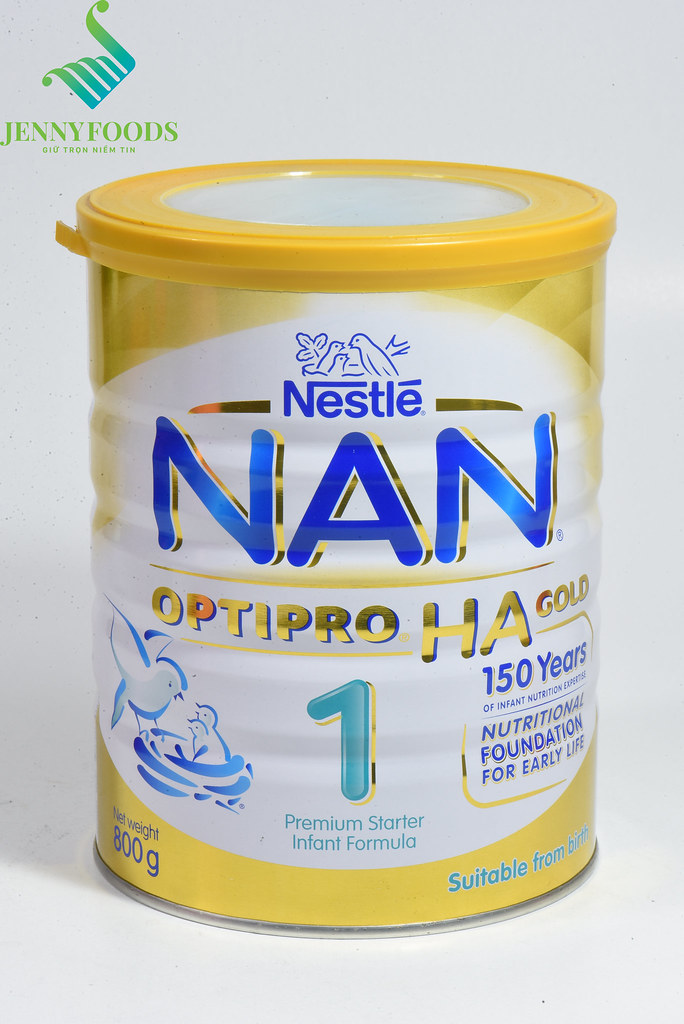This is a photograph of a tin can of baby formula against a white background. The can stands about seven inches high with a dark yellow lid featuring a white center that is resealable. The main background of the can is yellow, and it prominently displays a large white oval in the center, wrapping around its sides. At the top of this oval, in dark blue lettering outlined in gold, it says "Nestlé," with a blue Nestlé logo above it depicting a mother bird feeding baby birds in a nest. Below this, in large blue block letters with gold edges, it reads "NAN," followed by "OptiPro HA Gold" in gold text underneath. Dominating the center of the can is a large turquoise "ONE," labeled as "Premium Starter Infant Formula." To the right of this, in dark blue text, it states "150 Years Nutritional Foundation for Early Life." On the bottom left of the can, there is a depiction of a bird's nest with a mother bird feeding a baby bird. Additionally, the can mentions "800 grams" on the bottom left and "suitable from birth" on the right.